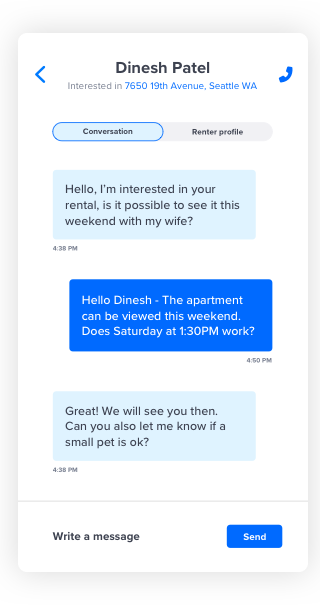**Screenshot Description:**

**Recipient: Dinesh Patel**

- **Text Alignment:** Centered
- **Font Color:** Black

**Message:**

- **Inquiry:** 
    - **Subject:** 7650 19th Avenue, Seattle, WA
    - **Message:** "Hello, I'm interested in your rental. Is it possible to see it this weekend with my wife?"
    - **Time:** 4:38 PM
    - **Background Color:** Dark Blue

**Response:**

- **Reply:** 
    - **Message:** "Hello Dinesh. The apartment can be viewed this weekend. Does Saturday at 1:30 PM work?"
    - **Time:** 4:50 PM
    - **Background Color:** Dark Blue

**Follow-up:**

- **Message:**
    - **Content:** "Great! We will see you then. Can you also let me know if a small pet is okay?"
    - **Time:**
    - **Background Color:** Light Blue

**Footer:**

- **Text Box:** "Write a message..."
- **Send Button:** Dark Blue Background with white text "Send" on the right side.